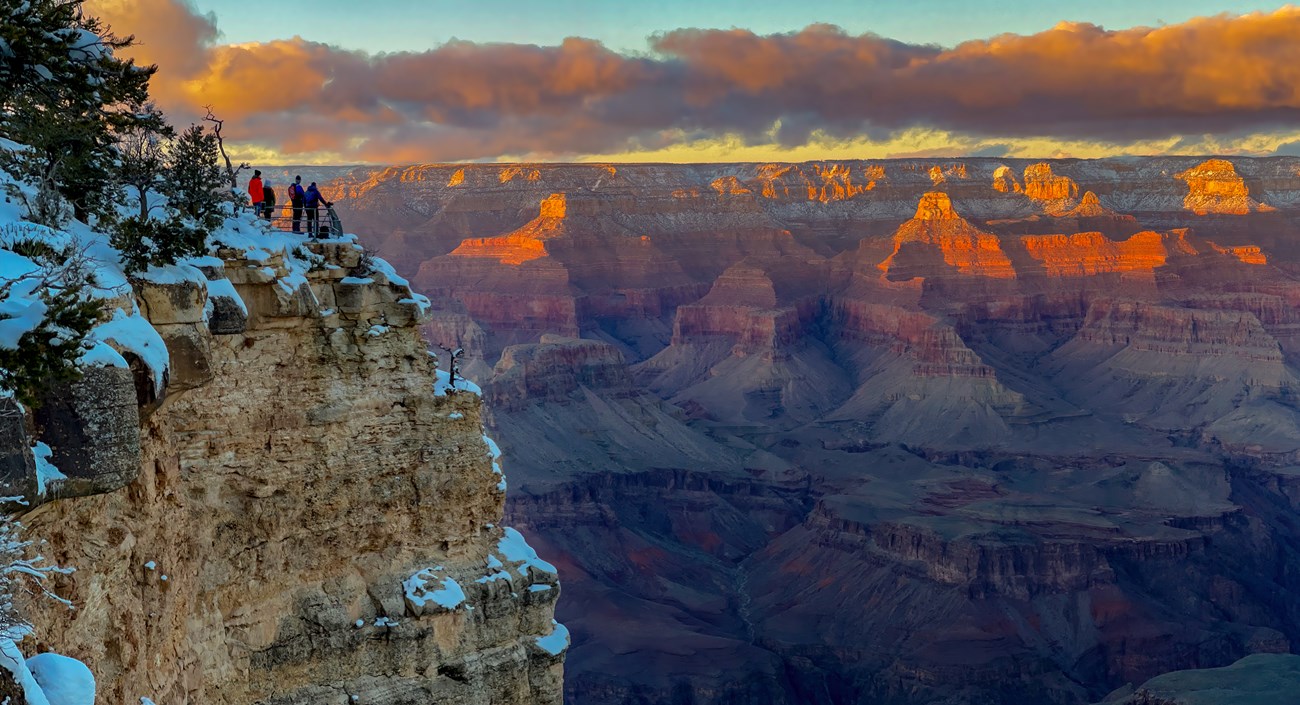This professional photograph captures a breathtaking winter sunset over the Grand Canyon. On the left side, a high mountain ridge, partially dusted with snow and accompanied by green trees, stands majestically. At the edge of this ridge, four hikers are visible from afar, dressed in distinct outfits: one in red, another in blue, and two in black. They appear to be intently gazing out over the expansive canyon below. The right side of the image reveals the Grand Canyon's vast, rugged interior, bathed in the soft, warm glow of the setting sun. The canyon’s sandy and rocky surfaces are illuminated in a vibrant palette of yellows, oranges, reds, and subtle purples and blues as the light fades. Above, the sky transitions from a dusky yellow-gray to a light blue, dominated by thick, orange-tinged clouds that enhance the scene's overall beauty.